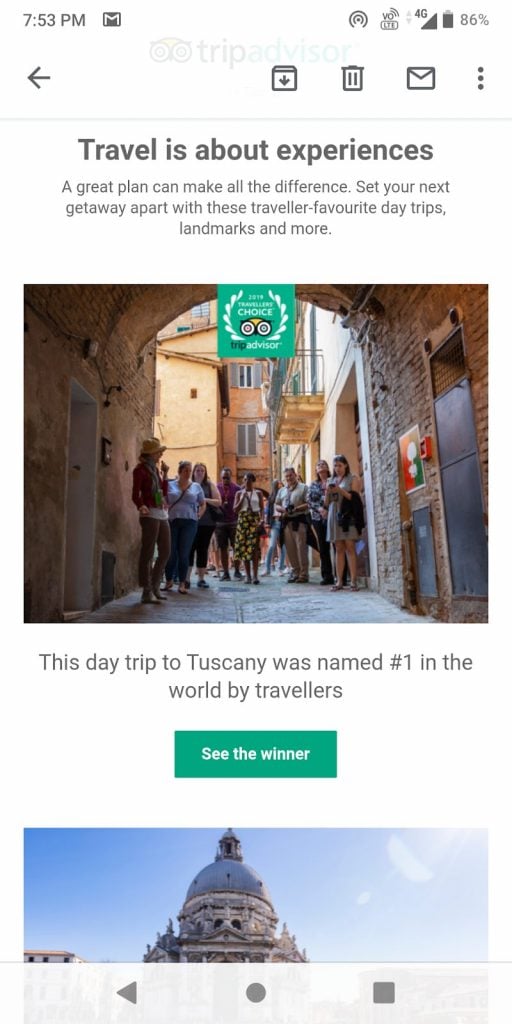This image showcases a mobile phone screen displaying a TripAdvisor webpage. The phone's battery life is at 86%, and it has a strong network connection. The current time displayed is 7:53 p.m. At the top of the screen, partially visible, are several icons: three vertically aligned dots, an envelope, a trash can, a download option, and a back arrow pointing to the left.

The webpage header reads "Travel is about experiences" in black font, with a subheading that states, "A great plan can make all the difference. Set your next getaway apart with these traveler favorite day trips, landmarks, and more." Below this text is a photograph of a group of people touring an ancient building, which appears slightly blurry.

Highlighted in green is a Choice Award badge, stating that a "Date trip to Tuscany was named number one in the world by travelers." A prominent green button labeled "See the Winner" is situated underneath this accolade. Additionally, there's a partially cut-off image of a mosque, peeking above a white band at the bottom of the screen which contains three icons. The overall layout and content emphasize TripAdvisor's recommendations for exceptional travel experiences.